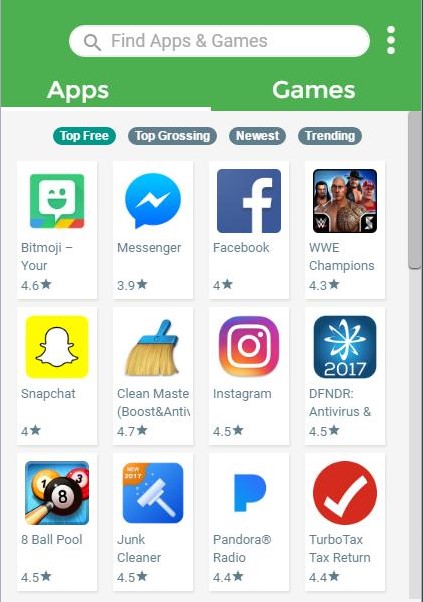This image is a detailed screenshot of a mobile app store interface. At the top, there is a green header bar with three horizontal lines on the left side, indicating a menu, and a search bar on the right side labeled "Find apps and games." Below the green header, the interface is divided into two main options: "Apps," which is currently selected and underlined in white, and "Games" on the right.

Directly underneath, there is a gray background with four filter buttons: "Top Free," "Top Grossing," "New & Trending," and "Top Free," which is currently selected and highlighted in green, while the others remain on a gray background.

The main content area displays three rows of app listings, each containing four vertically-aligned white boxes. Each box features an app logo, the app name, and its star rating out of five. The apps and their respective ratings from left to right, top to bottom, are as follows:

1. Bitmoji - 4.6 stars
2. Messenger - 3.9 stars
3. Facebook - 4.0 stars
4. WWE Champions - 4.3 stars
5. Snapchat - 4.0 stars
6. Clean Master (Boost and Antivirus) - 4.7 stars
7. Instagram - 4.5 stars
8. NDR Antivirus - 4.5 stars
9. 8-Ball Pool - 4.5 stars
10. Junk Cleaner - 4.5 stars
11. Pandora Radio - 4.4 stars
12. TurboTax: Tax Return App - 4.4 stars

The layout is clean and user-friendly, designed to facilitate easy navigation and discovery of new apps.